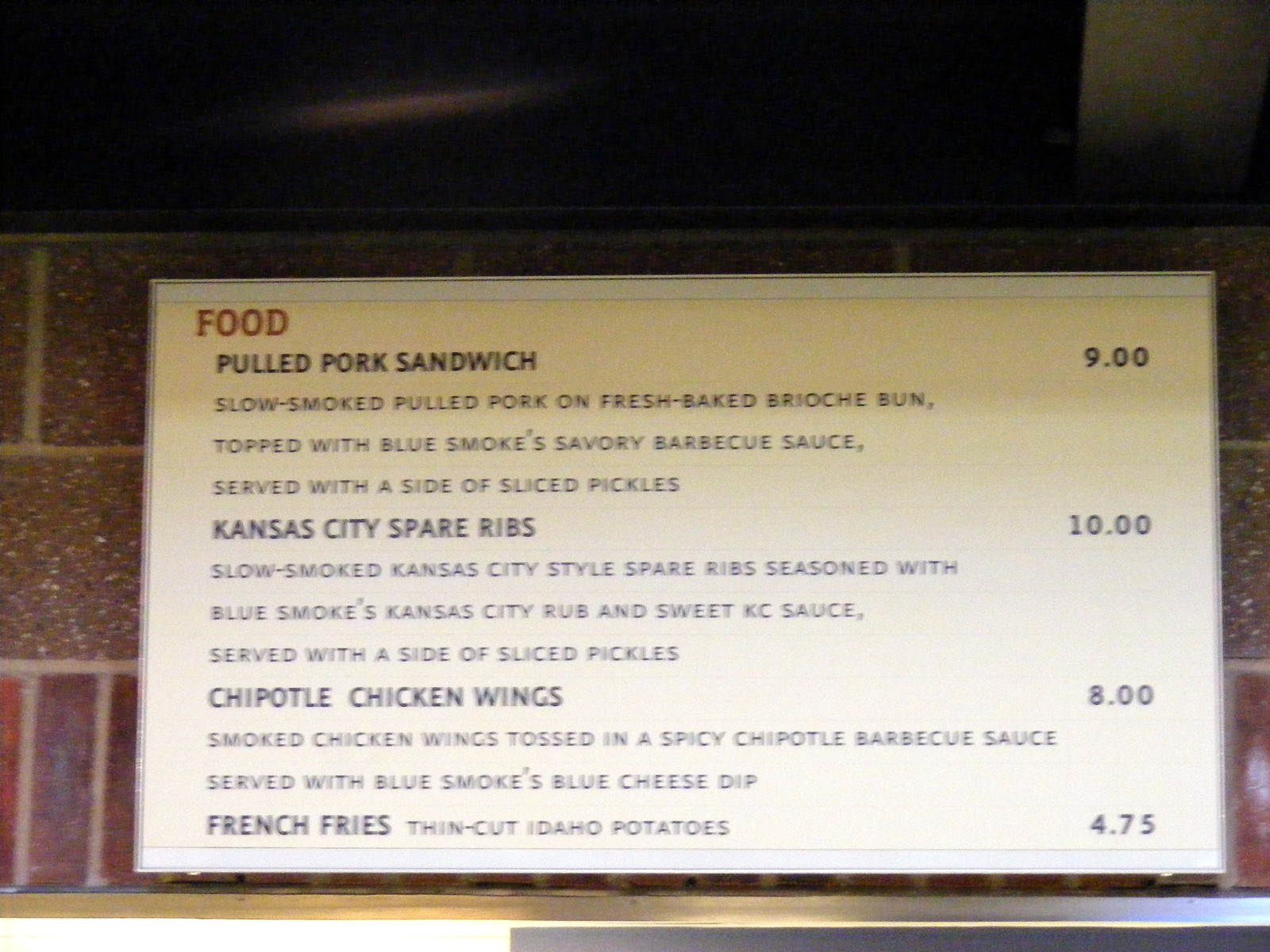A printed white sign is affixed to a brick wall, encased in a protective plastic frame. The sign prominently features a red heading labeled "Food" and lists several menu items in black text. Each dish is meticulously described, offering a mouth-watering selection:
  
1. **Pulled Pork Sandwich - $9:** Slow-smoked pulled pork served on a freshly baked brioche bun, topped with Blue Smoke's savory BBQ sauce and accompanied by a side of sliced pickles.
  
2. **Kansas City Spare Ribs - $10:** Kansas City-style spare ribs, slow-smoked and seasoned with Blue Smoke's Kansas City rub, finished with sweet KC sauce. Served with a side of sliced pickles.
  
3. **Chipotle Chicken Wings - $8:** Smoked chicken wings tossed in a spicy chipotle BBQ sauce, served with Blue Smoke's blue cheese dip.
  
4. **French Fries - $4.75:** Thin-cut Idaho potatoes, fried to perfection.

The repeated mention of "Blue Smoke" hints that the restaurant might be named after its signature BBQ sauce.